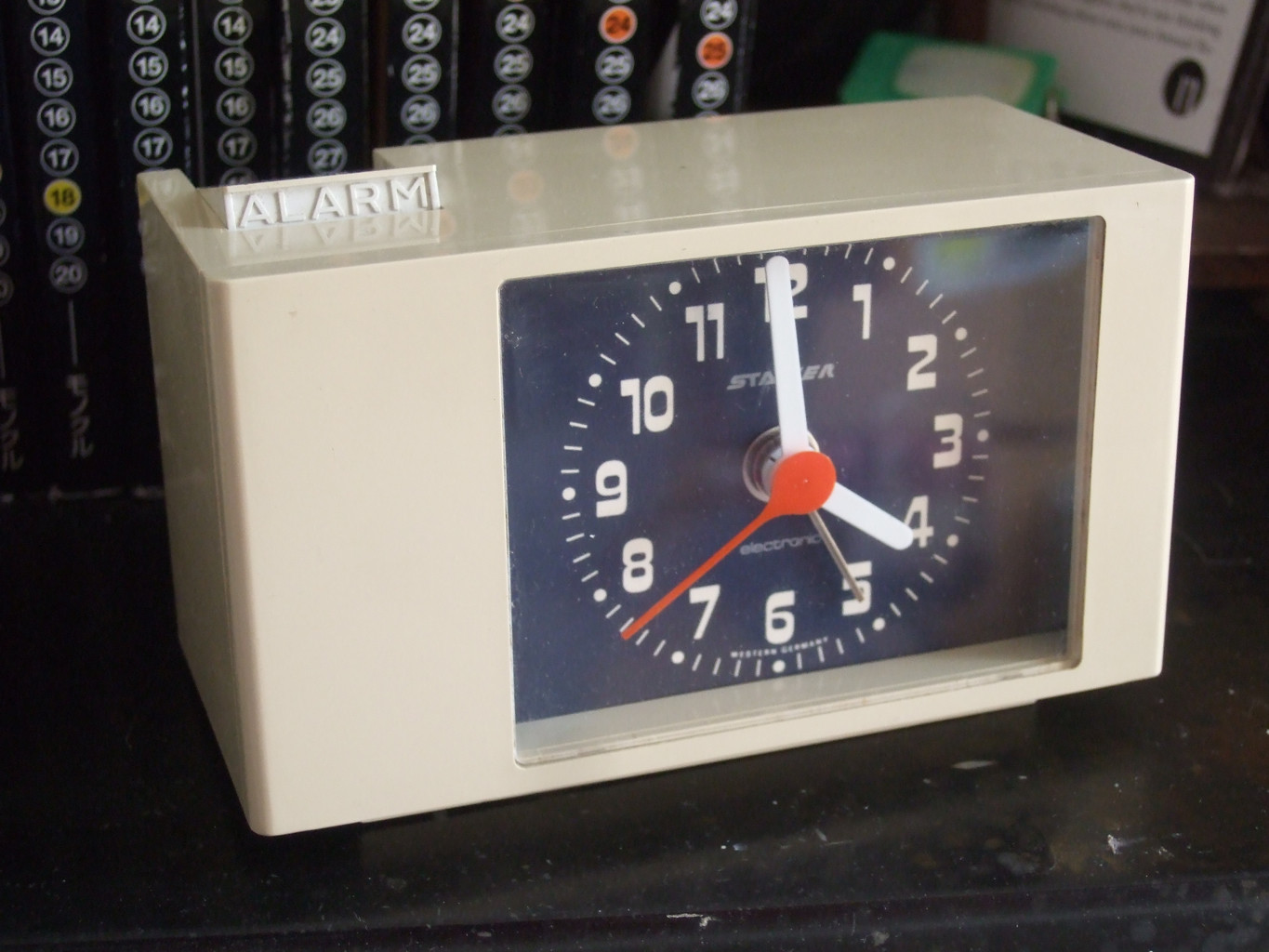This photograph captures a close-up view of a vintage rectangular alarm clock in a landscape orientation. The alarm clock has a distinctly aged and dated appearance, featuring a beige-colored exterior. Dominating the center of the clock is a black screen displaying white numbers, with the time set at 4 o'clock. This timepiece is positioned on a black table, situated at the top right corner from the viewer's angled perspective. In the background, several rows of circular number icons set against a black backdrop create a visually engaging contrast, each circle showcasing a number prominently in its center.